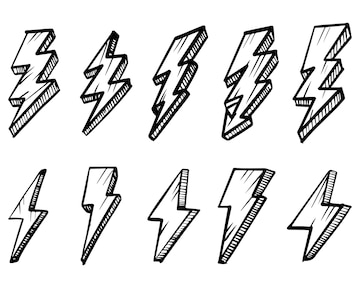The image is a black-and-white drawing featuring ten distinct lightning bolts arranged in two rows of five. The top row's lightning bolts are characterized by their three-segment, jagged appearance, with bold, shaded sides that give them a more dynamic, blocky, and cartoonish look. Notably, the fourth bolt from the left in the top row has a pointed arrowhead at the bottom. The bolts in the bottom row, each consisting of two segments, are shorter and simpler, resembling two connected triangles or rectangular shapes. Both rows display slight variations in shape, resembling clip art or comic strip illustrations, set against a plain white background.